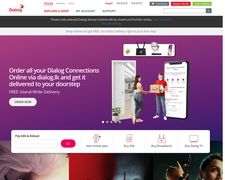A screenshot of a website shows a slightly blurry quality, particularly noticeable in the text at the top and bottom due to the small size of the image. The top section features a white border with a red logo, along with various options and buttons, including a search bar. Beneath this is a narrower black border with white text and a gray border with gray text, though the content of these sections is hard to decipher.

The central area of the screenshot is dominated by a purple background with prominent white lettering that reads: "Order all your digital connect or dialogue connections online via dialogue.jk and get it delivered to your doorstep." Below this text is an image depicting an open door. A young woman stands by the door, while a man in a red shirt is shown delivering something. Behind the man, an app interface on a cell phone is visible.